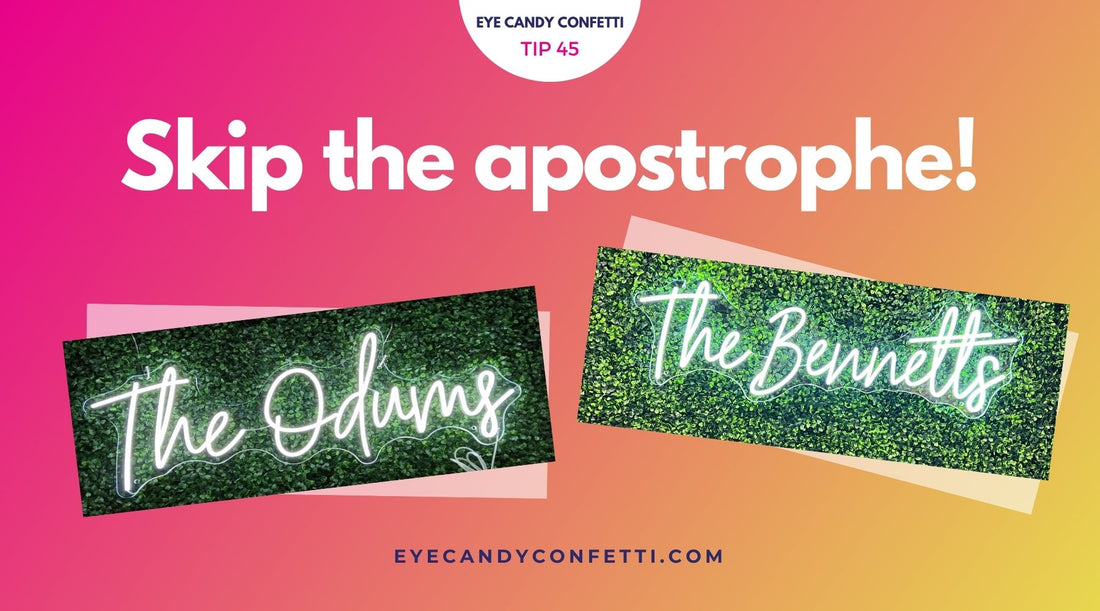This image is an advertisement with a scenic background that transitions from pink on the left to orange on the right. At the top, within a white, partially cut-off circle, black text reads "Eye Candy Confetti," followed by "tip 45" in dark pink. Below this, in white lettering, it boldy states, "skip the apostrophe!" Two rectangular photos dominate the center, both featuring green neon signs against a leafy backdrop. The sign on the left reads "The Otome," while the sign on the right displays "The Bennets," both presenting in green neon letters. The entire advertisement exudes a vibrant color gradient and concludes at the bottom with the website "eyehandyconfetti.com" in blue text.